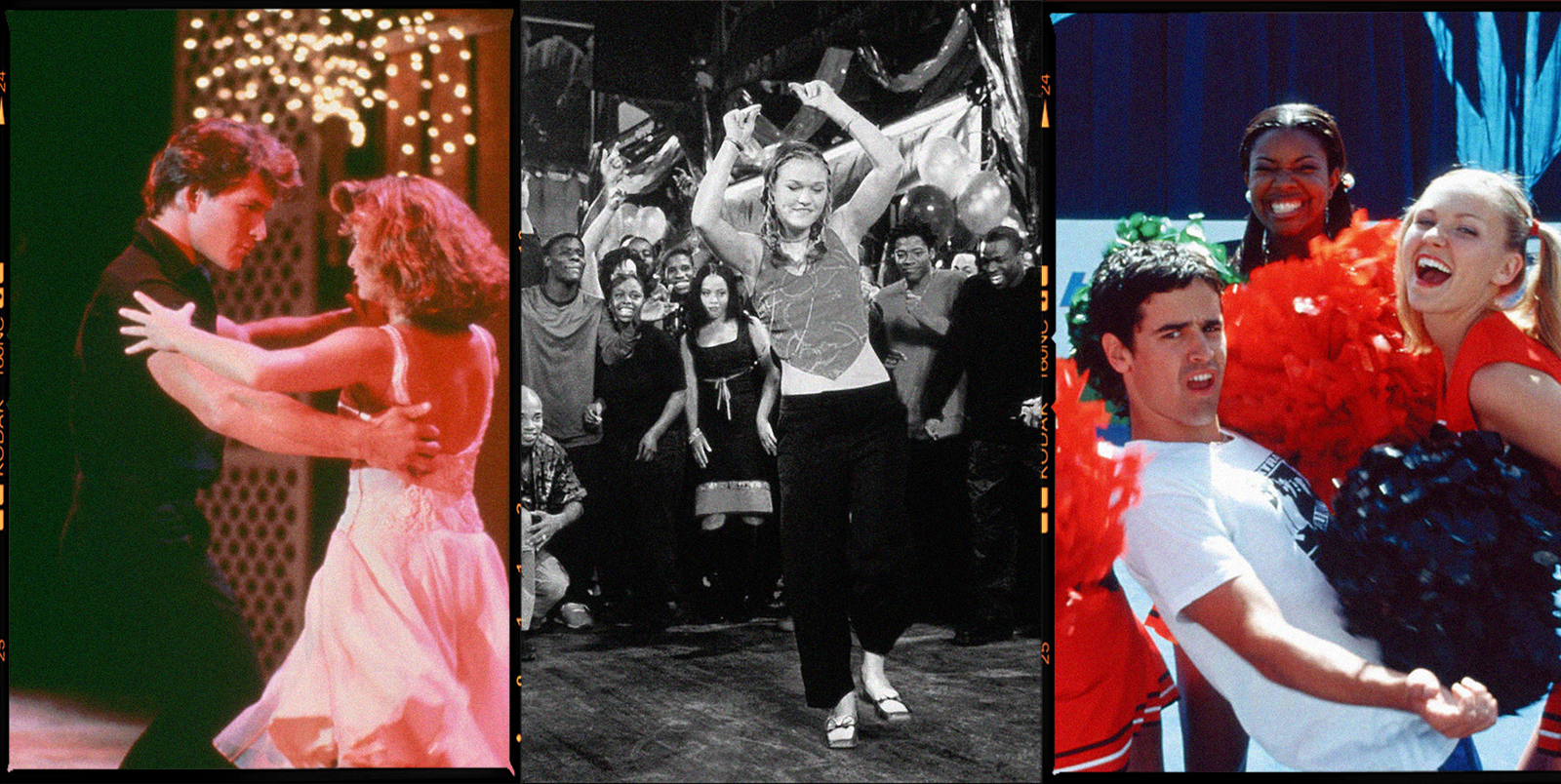This three-panel image features iconic scenes from different movies, each showcasing dancing in distinct settings. 

On the left, a scene from "Dirty Dancing" captures the film's main characters, a man in black dance attire and a woman in a white dress, intimately dancing outdoors under fairy lights, creating a romantic and nostalgic ambiance.

In the middle panel, a black-and-white image features Julia Stiles in what appears to be a scene from an early-2000s film. She strikes a confident pose with her arms raised, dancing amidst a crowd of onlookers who admire her performance.

The third panel depicts a lively moment from "Bring It On," showing three characters beaming with joy. Two cheerleaders in vibrant orange uniforms hold pom-poms, while a man in a white shirt leans back making a playful face. This image exudes a cheerful, high-energy vibe typical of high school cheerleading events.

Together, these images celebrate dance and youthful exuberance across different eras and cinematic contexts.